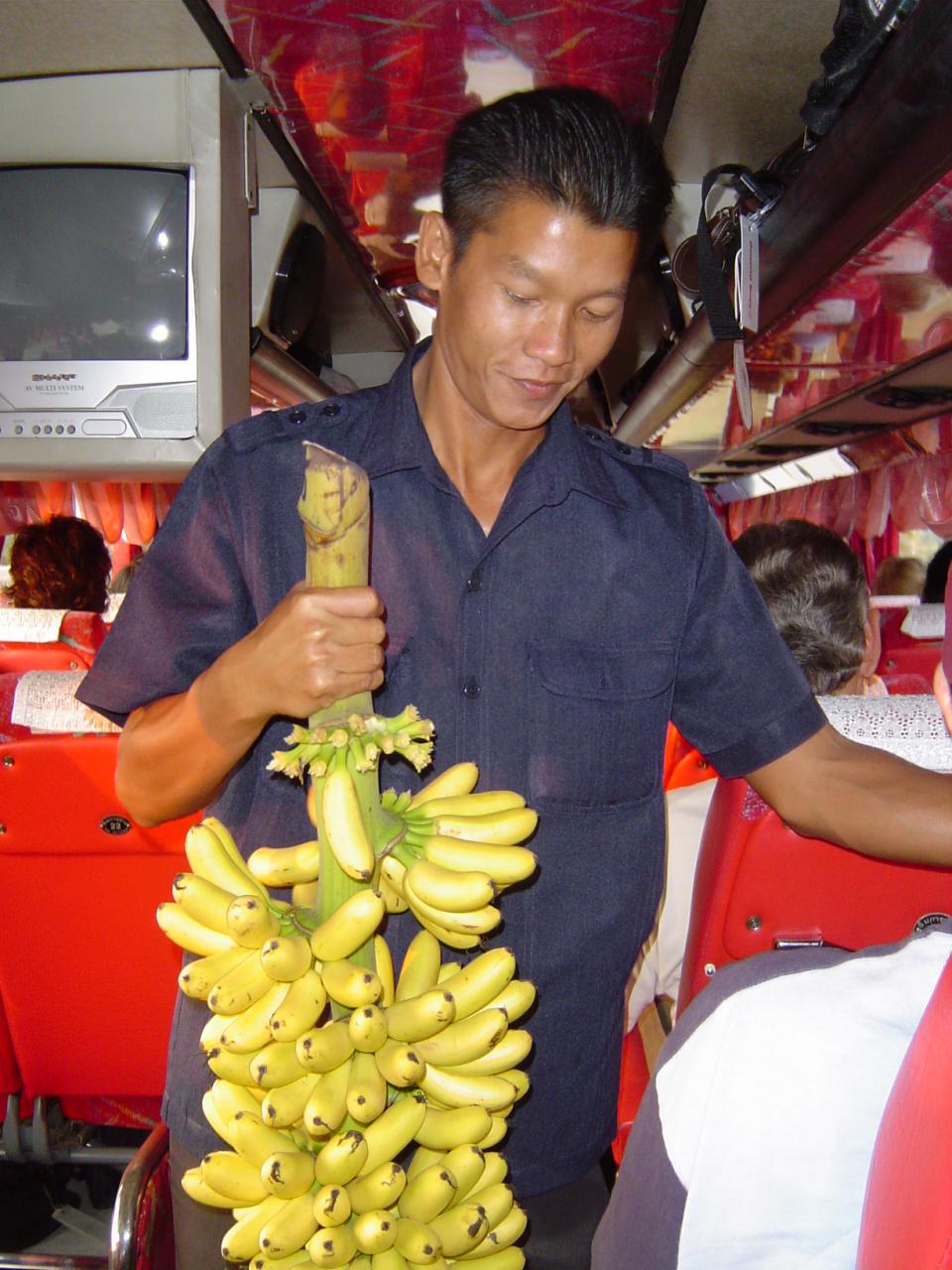The image depicts a man of likely Asian descent, standing confidently in the aisle of a bus with red and white seats. He has slicked-back black hair, tanned skin, and is dressed in a short-sleeved blue button-down shirt with a collar. The man is the central focus of the photograph, and he appears pleased, almost proud, as he holds a thick green stalk laden with small bananas that seem freshly cut from a tree. To his left, behind his shoulder, hangs an inactive silver TV screen, perhaps provided to entertain the bus passengers, whose heads are visible in the seats.